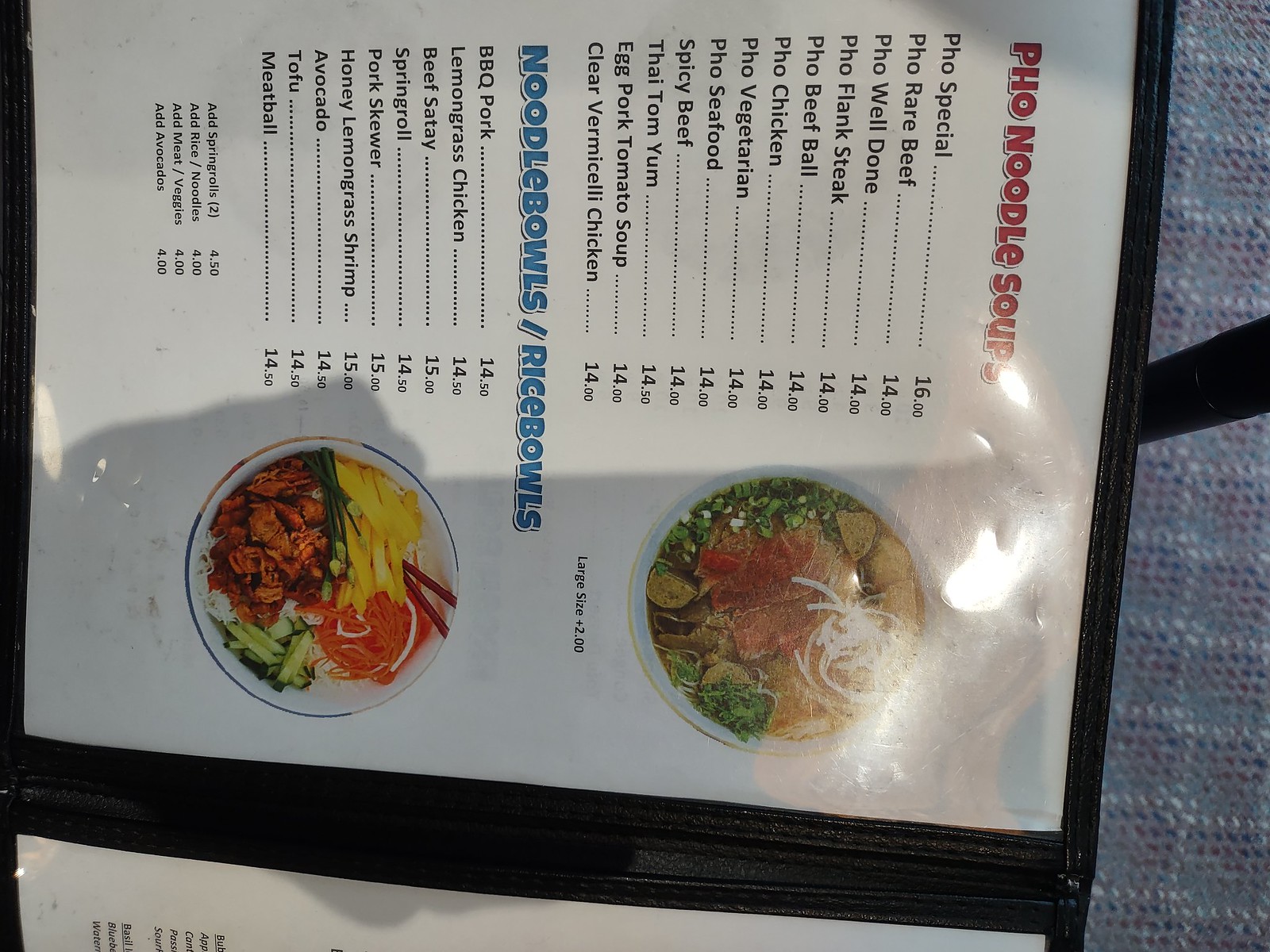In the image, a detailed food menu showcases a variety of Vietnamese dishes. At the top, the section titled "Pho Noodle Soups" features a list of different pho options along with their prices. Listed are:

- Pho Special: $16
- Pho Rare Beef: $14
- Pho Well Done: $14
- Pho Flank Steak: $14
- Pho Beef Ball: $14
- Pho Chicken: $14
- Pho Vegetable: $14
- Pho Seafood: $14
- Spicy Beef: $14
- Thai Tom Yum: $14
- Egg Pork: $14
- Tomato Soup: $14
- Clear Vermicelli Chicken: $14

To the right of this list, there is a picture of a steaming bowl of pho, emphasizing the dish's presentation and appeal. 

Below the pho section, another heading reads "Noodle Bowls/Rice Bowls." This section also includes images, with a picture of a rice bowl filled with savory ingredients on the right. The list of available dishes and their prices includes:

- Barbecue Pork: $14.50
- Lemongrass Chicken: $14.50
- Beef Steak: $15
- Spring Roll: $14.50
- Pork Skewer: $15
- Honey Lemongrass Shrimp: $15
- Avocado: $14.50
- Tofu: $14.50
- Meatball: $14.50

Each dish is neatly presented with clear pricing, making it easy for customers to select their desired meal. The menu's layout ensures that both text and images work together to provide a visually appealing and informative experience.